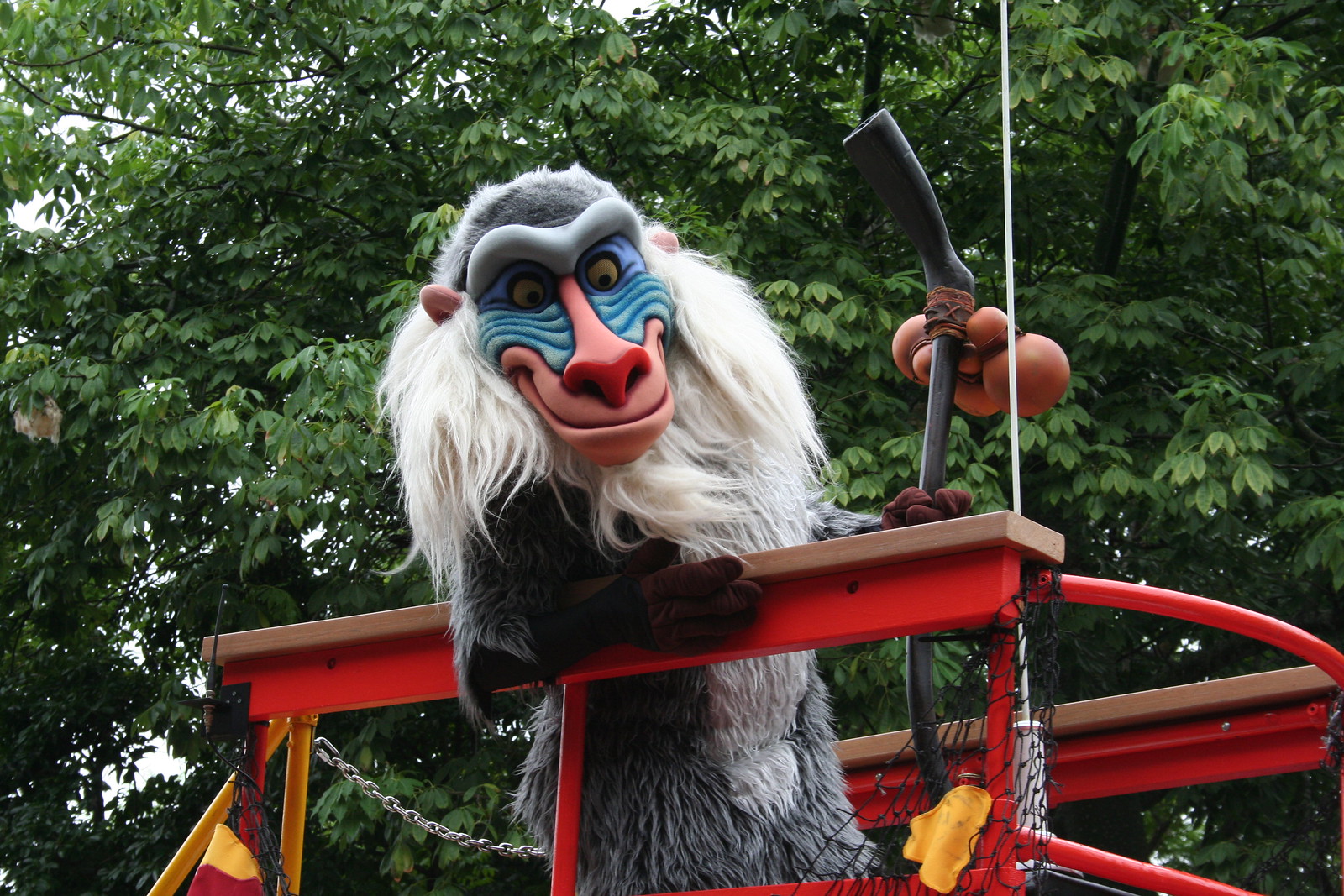This photograph, taken in landscape orientation, features a costumed character of Rafiki from Disney's "The Lion King" during a parade at Disney. The image captures Rafiki from the waist up, highlighting his distinctive features: a blue face, a large pink nose and mouth, small pink ears, and a wide pink smile. His facial appearance is complemented by a white beard that stretches from his ears down to his chin. Rafiki's body and arms are gray, consistent with his mandrill character design.

He stands on a vibrant red platform, holding a stick adorned with red items in his left hand. Rafiki appears to be looking down, adding a contemplative element to the scene. Behind him, a metal chain serves as a safety barrier, ensuring the performer remains secure on the platform. The background is lush with leafy trees, emphasizing the outdoor setting of the parade. The intricate details of Rafiki's costume, including the balls on the handle of his stick, and the evident safety measures, contribute to the overall engaging and celebratory atmosphere of the photograph.